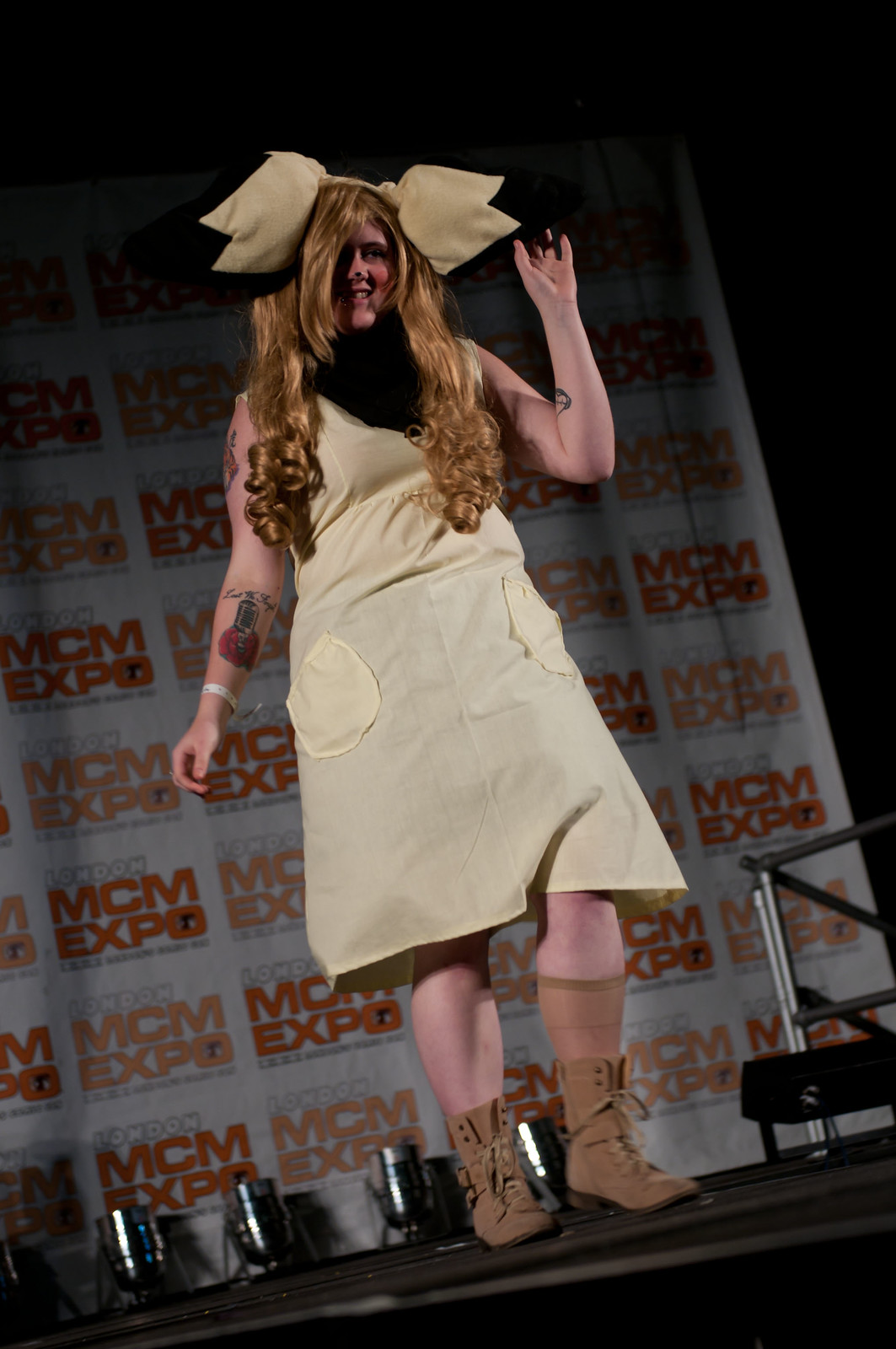The image is a photograph of a woman taken from a lower vantage point, giving an upward perspective of her standing on a solid black stage, likely at the London MCM Expo given the banner in the background with text reading "London MCM Expo" on a white background. The woman is wearing a sleeveless beige dress with hand pockets on either side near the waist, ending just below her knees. She completes her outfit with brown boots that have tan-colored laces, and a tan-colored sock on her left leg that reaches mid-calf. Her brown dyed hair, tied up with a large tan-colored bow resembling ears, cascades down her back. She has a tattoo on her underarm depicting a microphone on top of a red rose and a plastic wristband on her right wrist. The photograph captures a shadow under her chin, highlighting her poised presence on stage.